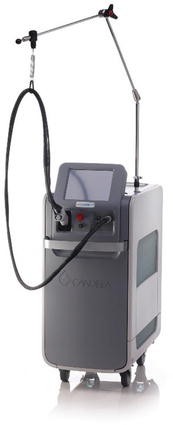The image depicts a medical device that resembles a portable, wheeled cart, standing about waist-high for an average male. The machine, primarily gray and white, has four wheels for mobility, emphasizing its portability. At the front top, it features a computer screen, connected via a black cable that is secured in two places beneath the screen. Directly underneath the monitor is a prominent red button. Extending from the top of the device is a long, articulating metal arm with at least two joints. This arm has a small hook at its end, suspending part of the black cable using a chain. Additionally, there are long antenna-like structures that contribute to holding up the cable or hose-like bands emanating from the cart, suggesting combined functionalities of both data monitoring and physical connectivity, likely necessary for medical applications. The overall appearance, with unique elements seldom seen outside of a hospital setting, suggests it could be employed in physical therapy or other specialized medical procedures.